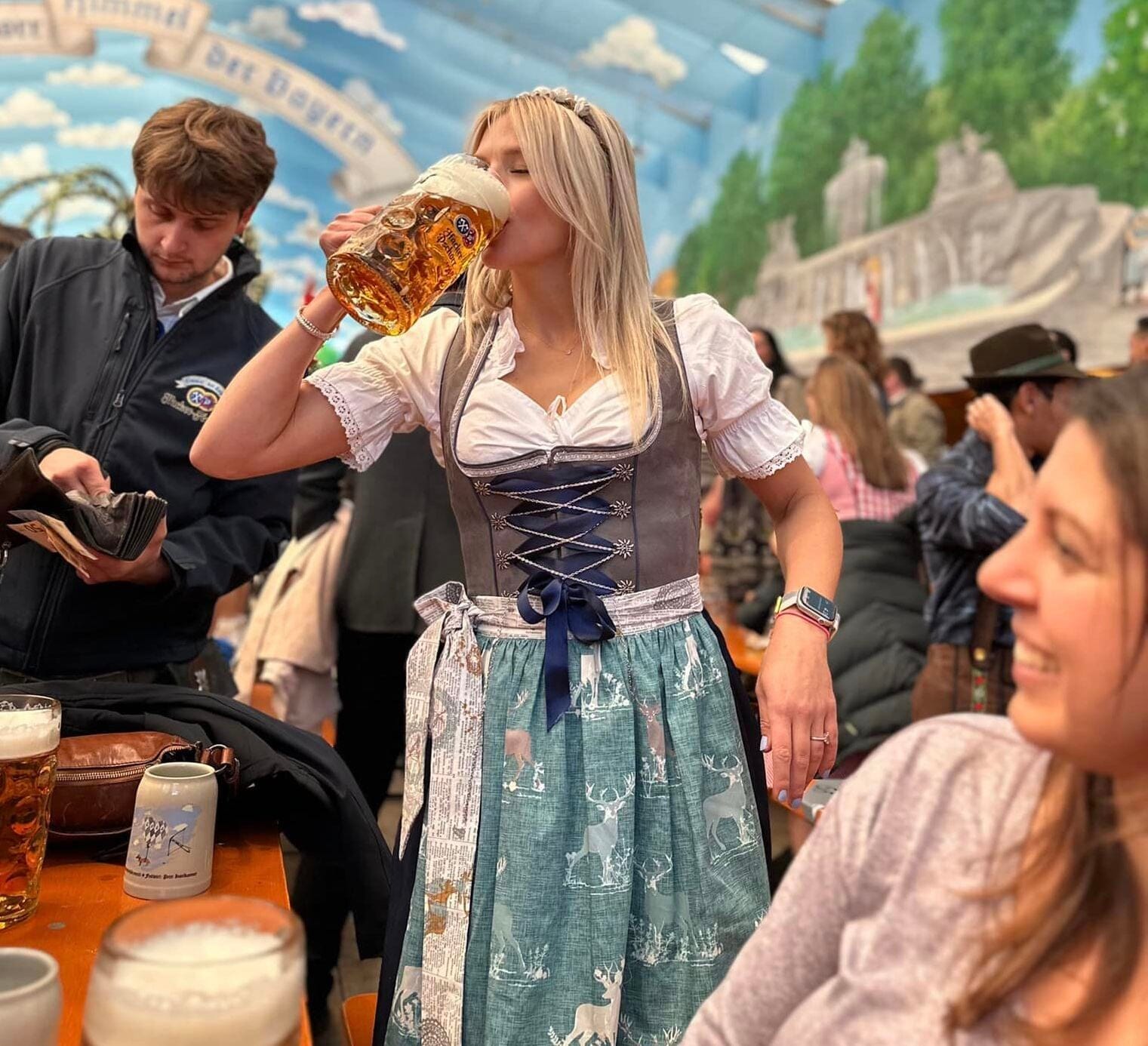This vibrant color photograph captures the lively atmosphere of what appears to be an Oktoberfest celebration. The focal point is a blonde woman adorned in traditional German attire— a laced-up corset over a white, frilly short-sleeved blouse and a light blue skirt patterned with deer. With her eyes closed, she lifts a large, frothy beer stein to her lips, savoring a sip. Her long hair cascades over her shoulders. To her left, a gentleman in a black jacket rummages in his wallet, possibly for cash. In the bottom right, a woman, although blurred, is visibly laughing, adding to the jovial mood of the scene. They are gathered around a wooden table that holds several glasses of beer and a metal beer stein with a design on it. The background is a mix of a crowd of people and a fantastical painted backdrop featuring a blue figure and a banner with German words, enhancing the festive ambiance.